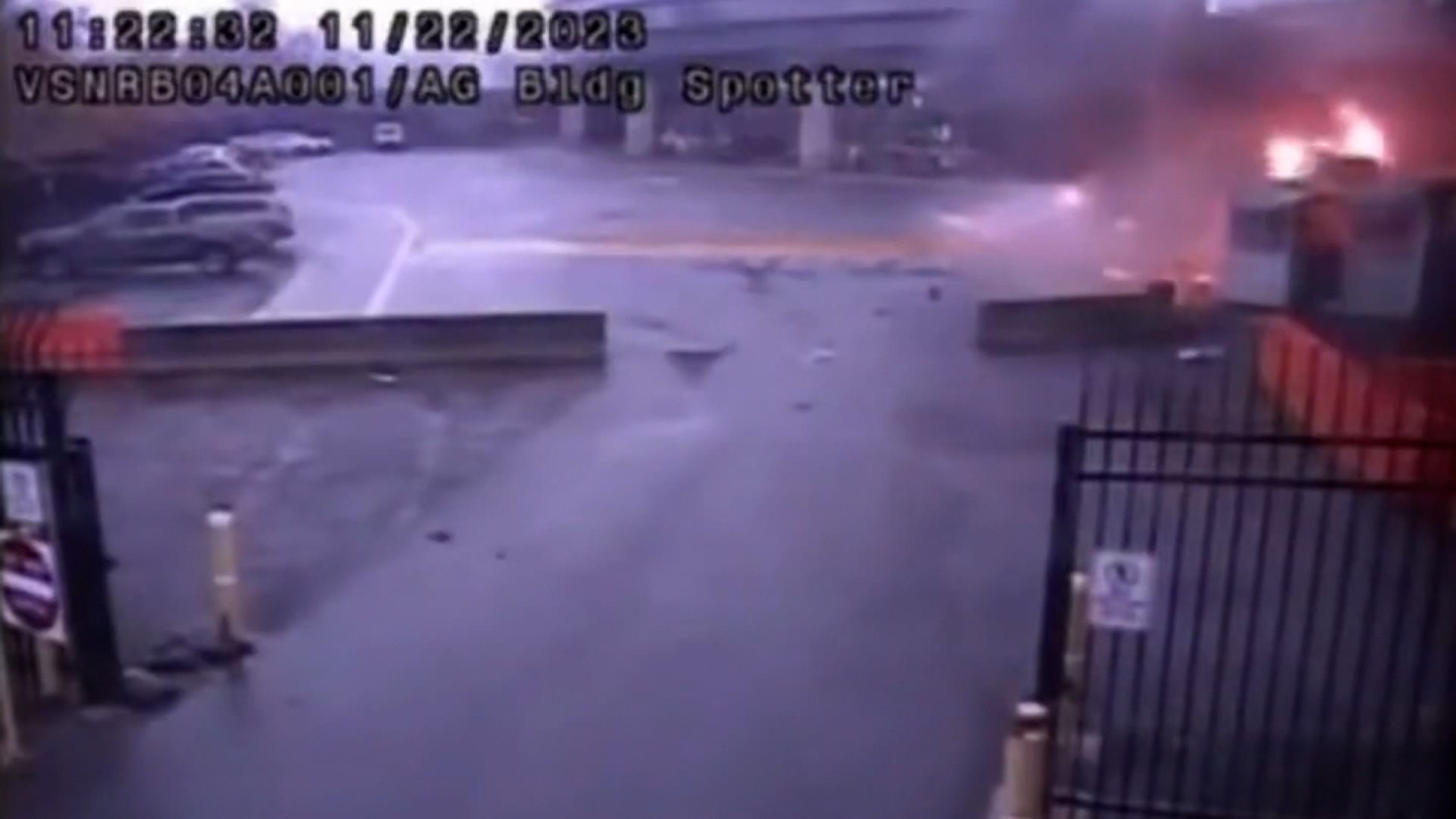The image captures what appears to be surveillance footage of a concrete parking garage, marked with the timestamp "11:22:32 11/22/2023" and labeled "DSNRB04A001/AG BLDG SPOTTER." In the upper left-hand portion, several cars are visible in parking spaces. The upper middle part of the image shows structural beams with cars parked on either side. To the upper right, an intense fire is evident with bright orange, yellow flames, and billowing smoke. Below the fire, on the right side, there's a small booth, next to a dark wall or barrier that partly extends into the left side of the image. The bottom left foreground shows the edge of a fence with a "Do Not Enter" sign, suggesting an entrance point below. On the bottom right, a black fence is visible with a white, unreadable sign, extending out of the frame. Notably, no people are visible in the image, suggesting it might be late at night when the fire began.